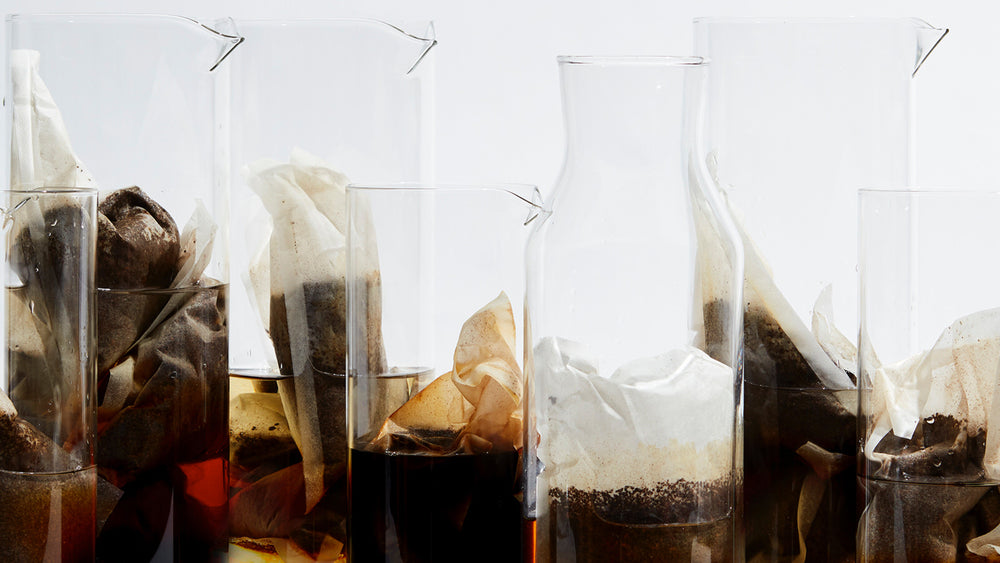The image features seven clear glass containers of varying shapes and sizes, lined up in two to three rows against a light background. Each container holds liquid, filled to about one-third to halfway up, with teabags steeping inside. The teabags vary in size and shape, with some being larger and appearing more like cloth sachets containing ground tea leaves. The containers include cylindrical glasses and ones with graduated tops that narrow, some featuring indentations for easier pouring. The liquid inside the containers shows varying degrees of steeping, producing shades of brown, white, orange, and red. Notably, the teabag in the bottom left container is steeping a reddish hue into the water. The arrangement shows the containers slightly overlapping each other, and the two at the ends are partially cut off in the image.